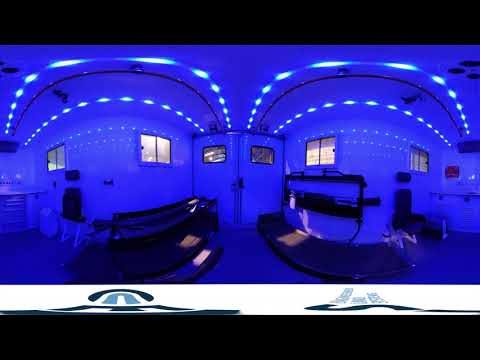The image depicts a room illuminated by a glowing blue light, creating an overwhelming blue ambiance throughout. The ceiling features white, upside-down U-shaped lights that give a semi-circular impression, possibly integrated onto curved surfaces. Prominent within the scene are central square windows, slightly illuminated and framed in black, positioned around eye level, about five to six feet from the floor. A noticeable black horizontal line runs across the image, reinforced by another parallel black line underneath it. Below the windows on the left, there are some rectangular objects which could be interpreted as either black squares or cases on wheels, while an adjacent black rectangle might be a counter winding its way leftward. Towards the right of the image, what appears to be a mat extends from the corner towards the center. The overall reflective quality of the room along with the curved tables and possibly a door suggests a highly mirrored, almost distorted three-dimensional space, hinting at an exercise or music studio. Despite the dominant blue coloration, the precise function of the room is hard to determine, amplified by the mirrored, exaggerated reflections.